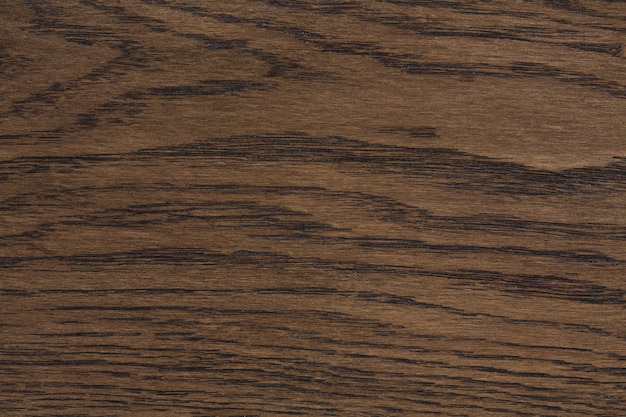The image is a close-up of a medium-toned wood grain surface, likely paneling, with a rich, horizontal grain pattern. This pattern features varied grain lines, including darker, curved lines predominantly concentrated towards the top left of the image. These lines become less curved and more tightly spaced as they descend, especially towards the bottom where they run straighter and closer together. A noticeable notch is present around the middle of the image, slightly to the left. The grain, which might belong to a heavily stained oak or possibly walnut, exhibits a mix of wide, smooth areas and fine, dark bands, forming an intricate and detailed wood texture across the entire frame.